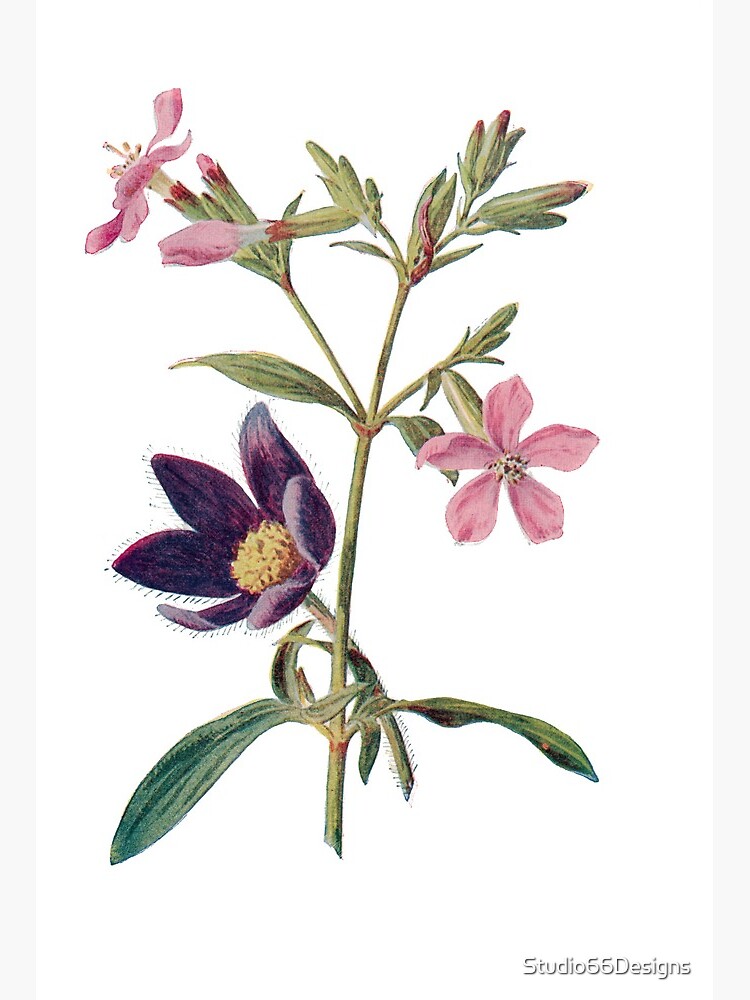This detailed illustration, resembling a scientific drawing in the Audubon style, features a stem of a flowering plant on an off-white background, labeled "Studio 66 Designs" at the bottom right. The main stem branches out, displaying a lifelike and clinically precise representation of various stages of blooming flowers and foliage. 

At the top left branch, a fully bloomed, pink flower with a whitish red center showcases four visible petals. Just below, on the same branch, another pink flower is in mid-bloom next to a pink bud. On the right, two buds remain unopened, hinting at future blossoms.

Descending toward the stem's base, to the left, there's a captivating rich purple flower with a yellow-orange center, surrounded by a delicate fuzziness. Adjacent to these blossoms are several leaves, ranging from blue-green to darker hues, some drooping gently downwards. This botanical illustration captures both the beauty and the minute details of plant life, making it an exquisite and educational piece.